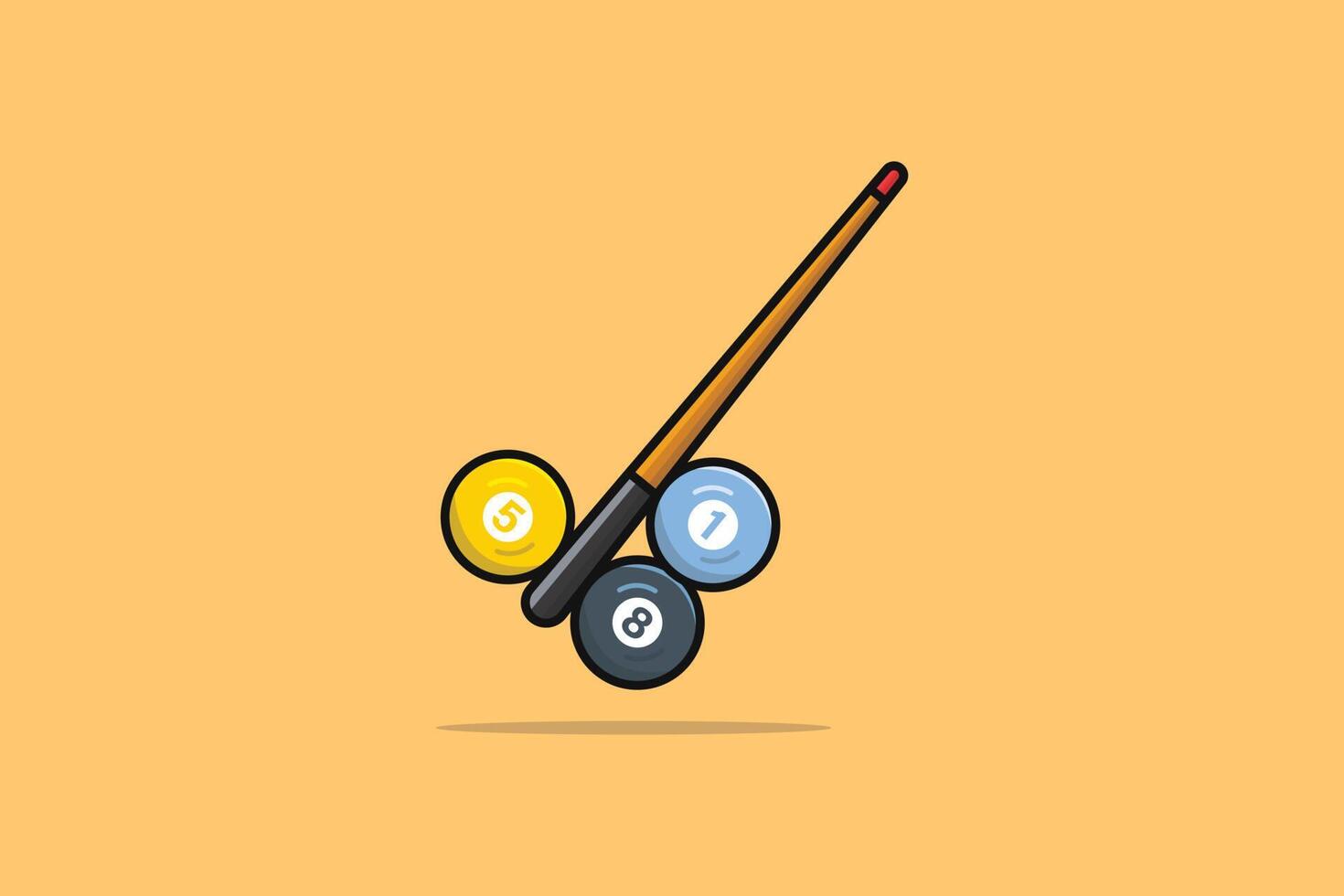This is a detailed art illustration of a billiard scene set against a golden yellow, almost cartoonish background. The focus is on a vertically angled billiard cue stick and three prominently displayed billiard balls. The cue stick starts with a dark black handle at the bottom, followed by a brown wooden section, leading to an orange area just before it culminates in a red pointed tip. The stick points upwards to the right, creating a dynamic composition.

Near the base of the cue stick is the yellow number 5 ball, with a white circle and the number 5 inscribed within it. Directly adjacent to the black handle of the stick is the solid black number 8 ball, which also features a white circle and a black number 8. Positioned slightly higher and almost under the stick, you find the baby blue number 1 ball, marked similarly with a white circle and the number 1. The arrangement gives a sense of the balls being in motion, suspended in midair, creating a vibrant and dynamic scene typical of a graphic illustration. The vibrant colors and the scale of the balls in relation to the stick add a playful, almost surreal touch to the artwork.